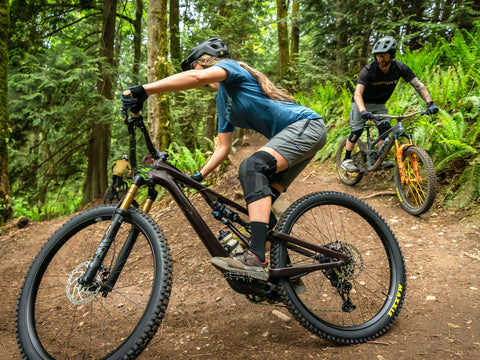In an outdoor setting, this detailed image captures a vibrant scene of mountain biking on a dirt trail winding through the woods. Tall trees and lush ferns adorn the forest floor, creating a picturesque backdrop. Dominating the foreground is a young woman in a teal-colored shirt and gray shorts, skillfully navigating a sharp turn on her black mountain bike, which features deep-tread tires designed for off-road cycling. Her long hair flows beneath a black helmet, and she wears black knee pads, hand gloves, and gray shoes. Her face is obscured, adding a sense of anonymity and focus on her athleticism. Just behind her, a young man on a similar type of bike - possibly a mountain bike or BMX - follows suit. He is dressed in a black t-shirt, gray shorts, knee pads, gloves, and a gray helmet. The composition captures the thrill and intensity of mountain biking amid the captivating natural beauty of the forest trail.